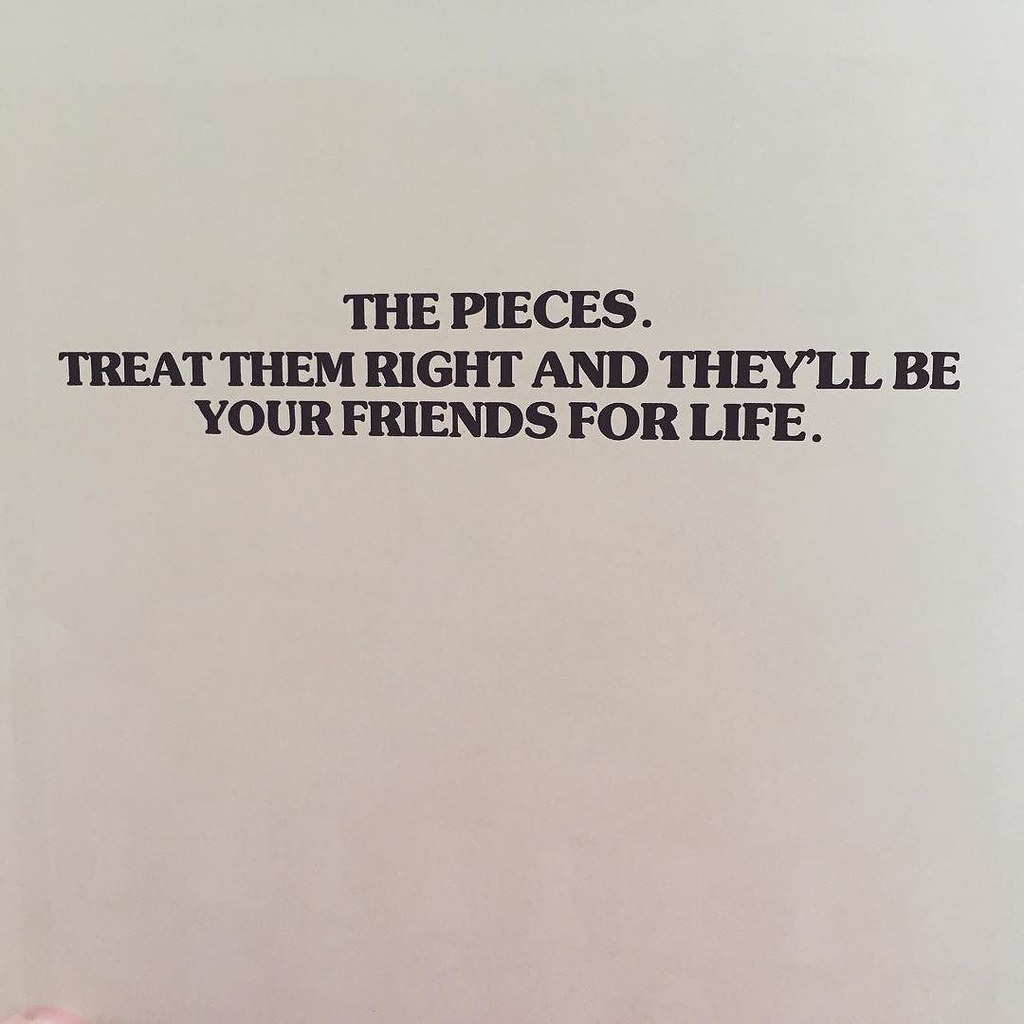The image is a square photograph depicting a slightly grayish, possibly shadowed, surface that is either a piece of paper or a wall. Positioned slightly above the center are three lines of bold, black text. The quote reads, "The pieces. Treat them right and they'll be your friends for life." The text is center aligned and the excessive punctuation emphasizes the importance of "the pieces," possibly referring to aspects of life. The overall scene is minimalistic, with the focus entirely on the text. There is a slight reddish discoloration in the bottom-left corner, suggesting the paper might have gotten wet, adding a small, almost unnoticeable imperfection to the otherwise blank background.